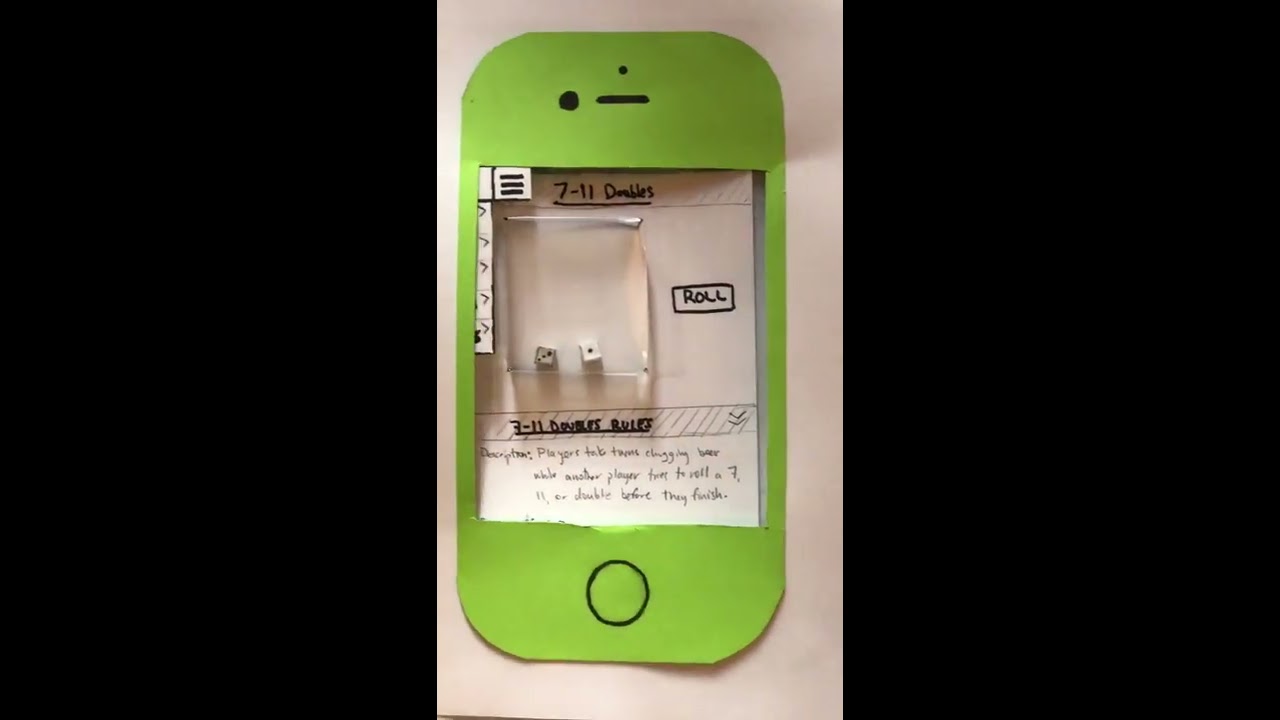This is a detailed photograph of a handcrafted lime green paper cutout resembling a smartphone, centered on a beige background. The cutout mimics the appearance of a modern iPhone, complete with a black circular switch button and black designs that suggest a camera and speaker at the top. The screen area is depicted in white, featuring handwritten text that reads "7-11 Doubles" at the top. Below this title, there are two small dice displayed, one showing the number three and the other displaying one. To the right of the dice, there's a black rectangle with the word "roll" inscribed. Further down, a segment of text titled "7-11 Doubles Rules" is also handwritten, describing a drinking game where players tag-team chugging beer while another player attempts to roll a 7, 11, or a double before they finish. The left side of the cutout includes a small piece of paper with three black lines drawn on it, resembling a menu button. The entirety of the cutout is bordered by black tape or borders on both sides, and the focus of the photo is solely on this intricately designed paper phone.